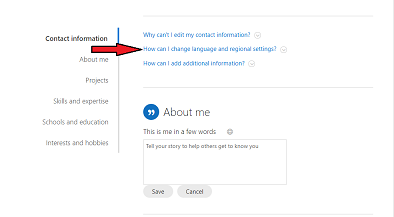This image showcases a webpage with various navigational tabs and a prominent contact information section. The page features five vertical tabs on the left side, listed from top to bottom: "About Me," "Projects," "Skills and Expertise," "Schools and Education," and "Interests and Hobbies." 

In the main white section of the webpage, which contrasts with sky-blue text, there is a central question posed: "Why can't I edit my contact information?" Directly beneath this, a red arrow points to the right, accompanied by the text, "How can I change language and regional settings?"—indicating the user's interest in modifying these preferences.

Further down, the page provides additional guidance with the question, "How can I add additional information?" followed by a section labeled "About Me." This section invites the user to share personal details with a text box under the prompt, "This is me in a few words." The accompanying text encourages users to, "Tell your story to help others get to know you," with options to either save or cancel their input.